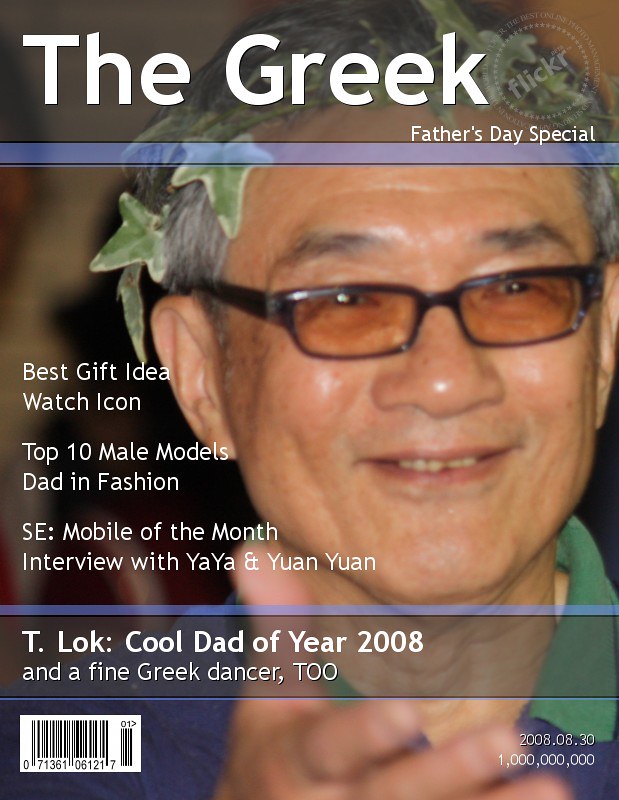The magazine cover titled "The Greek," features an older Asian man, presumably around 60 years of age, prominently positioned from the chest up. He is donning rectangular, thick-rimmed glasses with tinted orange-reddish lenses and has a slight, pleasant grin on his face. His hair, tinged with gray, is adorned with an ivy wreath reminiscent of a classical toga party. The man is dressed in a polo shirt with a green collar, the body of the polo appearing blue, and his right hand is visible and outstretched at the bottom of the photo. 

In white font at the top-left, the title "The Greek" is displayed, with "Father's Day Special" immediately below it. To the left of the man's face, several text lines provide content highlights, including: "Best Gift Idea," "Top 10 Male Models: Dad in Fashion," "SE: Mobile of the Month," and "Interview with Yaya and Yuan Yuan." Within a shadowy horizontal strip at the bottom, the text reads: "T-Lock: Cool Dad of the Year 2008 and a Fine Greek Dancer TOO." A black and white barcode is present at the bottom-left corner, while the date "2008.08.30" and the number "1,000,000,000" are printed in very small white text at the bottom-right. Additionally, a faded circular Flickr watermark is located at the upper right corner.